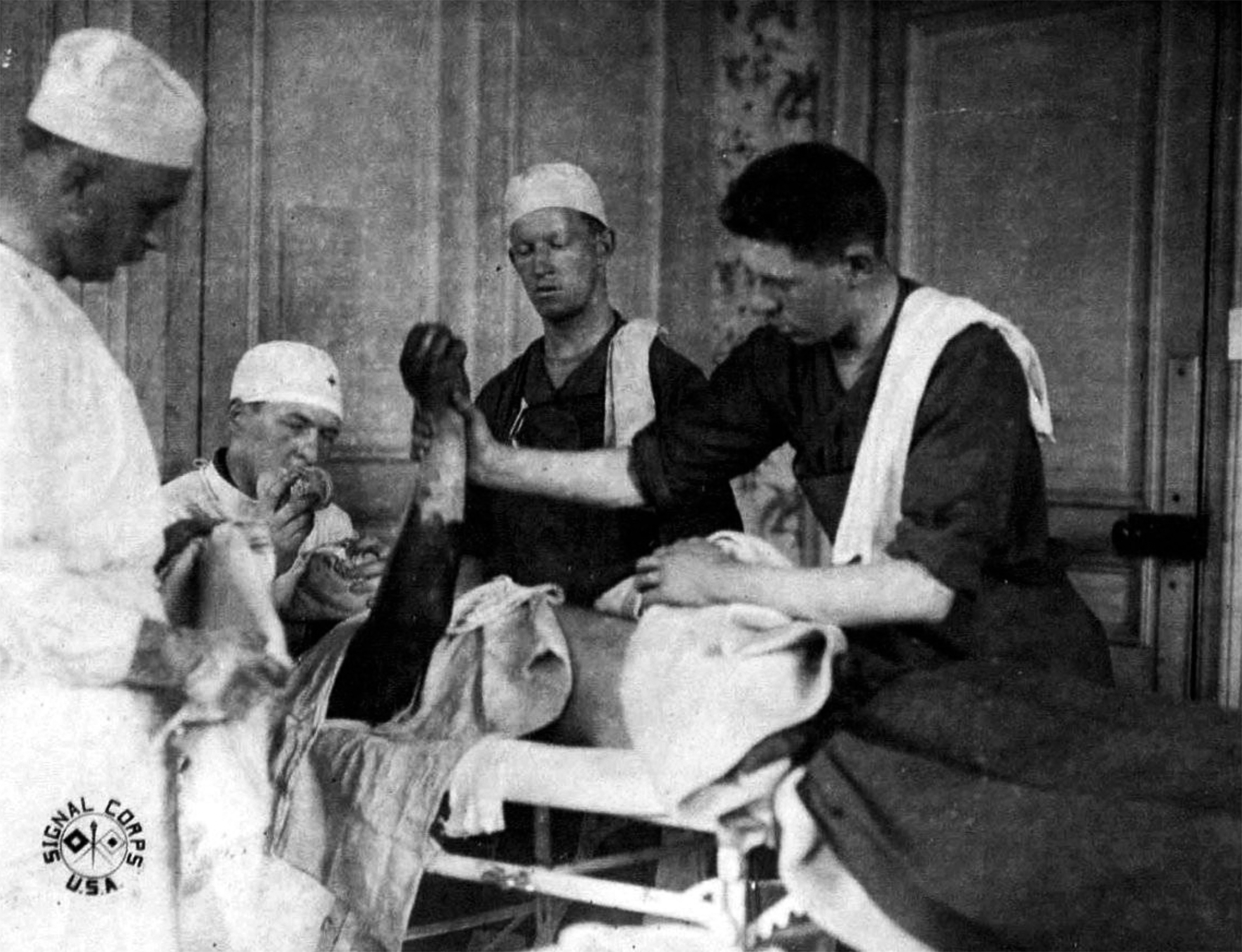This black-and-white photograph captures a somber scene in what appears to be a makeshift surgical room, possibly from a wartime or emergency setting. At the center of the image lies an injured male patient on a rudimentary hospital bed or stretcher, draped partially with a blanket. His right arm, appearing severely charred or burnt, is raised by a medical professional, revealing dark, damaged skin with a contrasting lighter area where the person's hand grips it. The patient is also wearing a peculiar vest that is only attached by one sleeve. 

Surrounding the patient are multiple individuals, likely doctors or surgeons, deeply engrossed in their tasks. One of them is positioned at the patient's head, seemingly tending to his face or mouth. Another person stands facing the right side of the picture in a white uniform with a cap, hinting at their medical role. In the background, two figures clad in black outfits with white surgeon's caps are also present. Each of these individuals has a towel draped over their shoulders, possibly indicating their involvement in the ongoing medical efforts.

This powerful image, marked "Signal Corps USA" in the lower left corner, underscores the intense and critical nature of the situation, emphasizing both the urgency and the collaborative effort of the medical team.